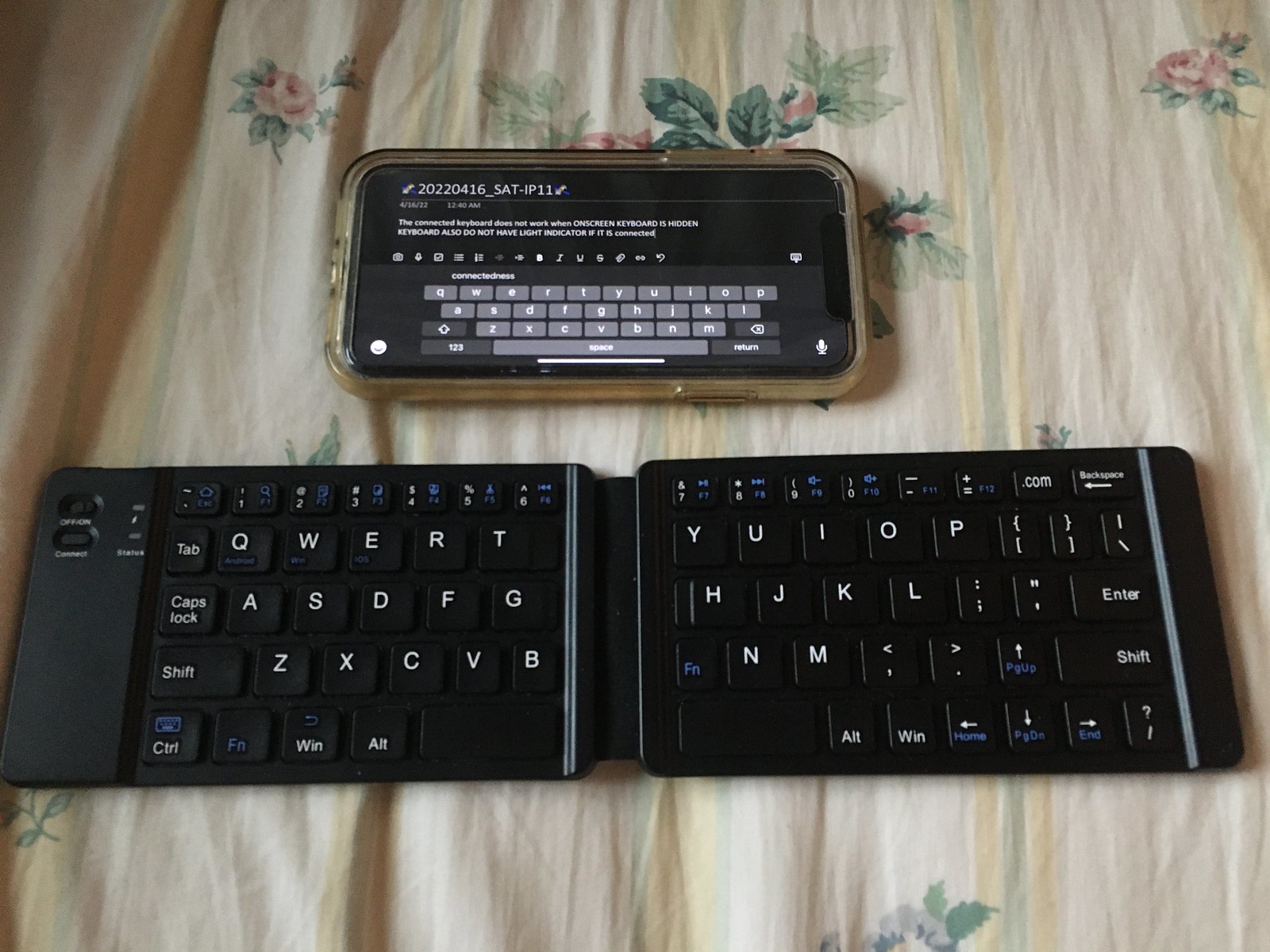Displayed on a vintage-style, floral-patterned tablecloth with pale yellow and green stripes, an image showcases an older model iPhone and a foldable, QWERTY-style keyboard. The tablecloth is off-white with pink and off-white flowers and green leaves, lending an old and somewhat disheveled appearance to the scene. The iPhone, encased in a transparent amber case, displays a note with text indicating that the connected keyboard will not function when the on-screen keyboard is hidden and lacks a connection indicator. The note also contains a potential date and time, "April 16, 2022, 12:40 a.m." The portable keyboard, black and thin, is folded out to reveal the entire layout, split at the T, G, and B keys. Both the keyboard and the phone appear to be relatively new and are likely connected via Bluetooth.